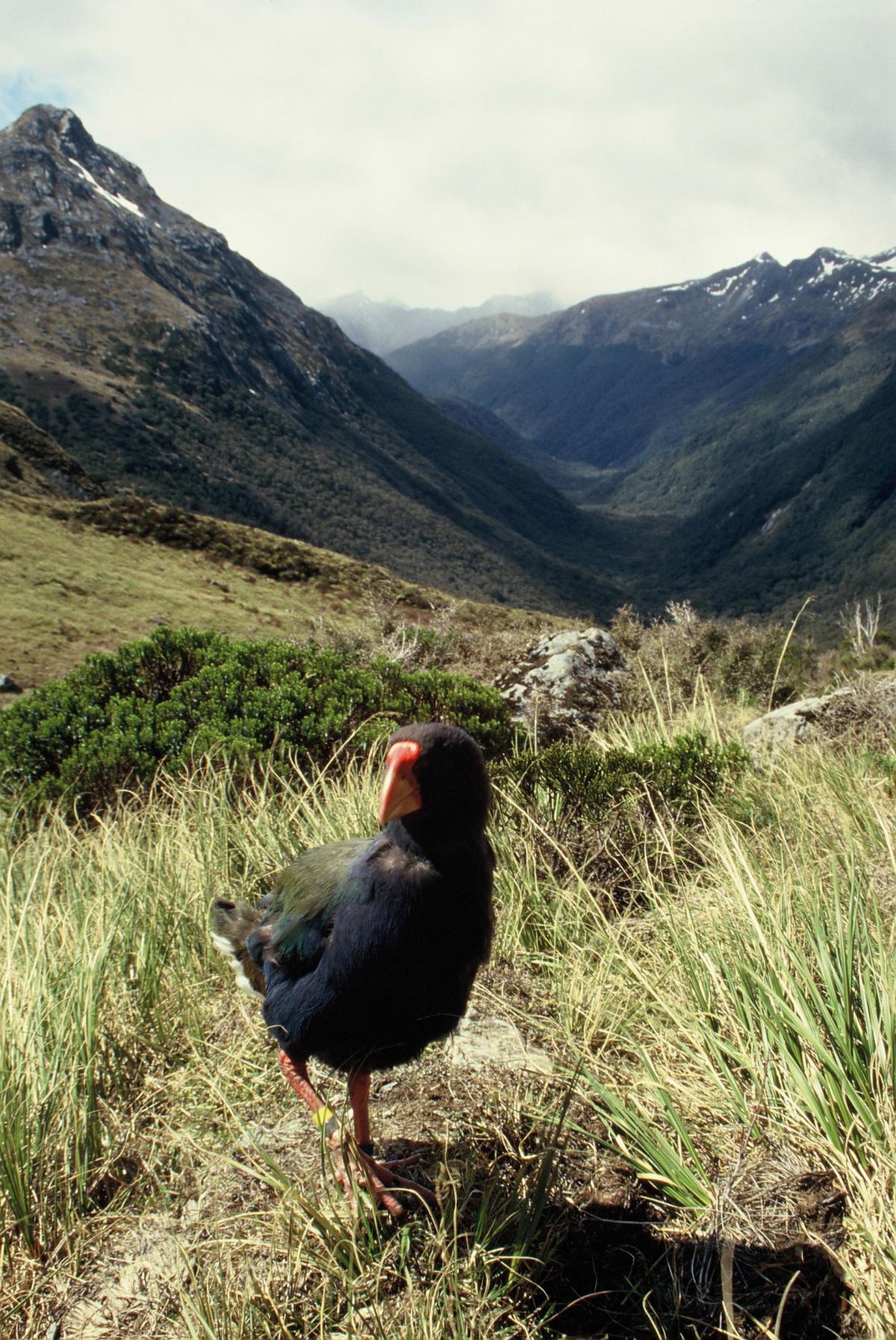In this carefully detailed photograph, a strikingly colorful bird is captured standing in a grassy field within a mountainous area. The bird, notable for its unique color palette, stands prominently on one orange leg, gazing to the left. Its beak is similarly orange but shows a hint of red at the top. With a dark plumage that reveals hints of blue, teal, and green, the bird's belly is distinctly blue while the upper parts transition into green and gray tones.

The scene is set against a backdrop of a vast, snow-capped mountain range that stretches across the horizon. The peaks are shrouded in fog, indicative of a cloudy day. Adding to the picturesque nature of the setting is a verdant valley nestled between the mountain ranges, characterized by its darker green foliage which contrasts with the foreground's lighter-colored tall grass, moss, and scattered rocks.

The crisp detail with which the bird and the landscape are depicted gives a vivid sense of the serene yet dramatic environment, where a clear sky meets imposing natural features, and the vibrant bird adds a touch of liveliness to the secluded meadow.